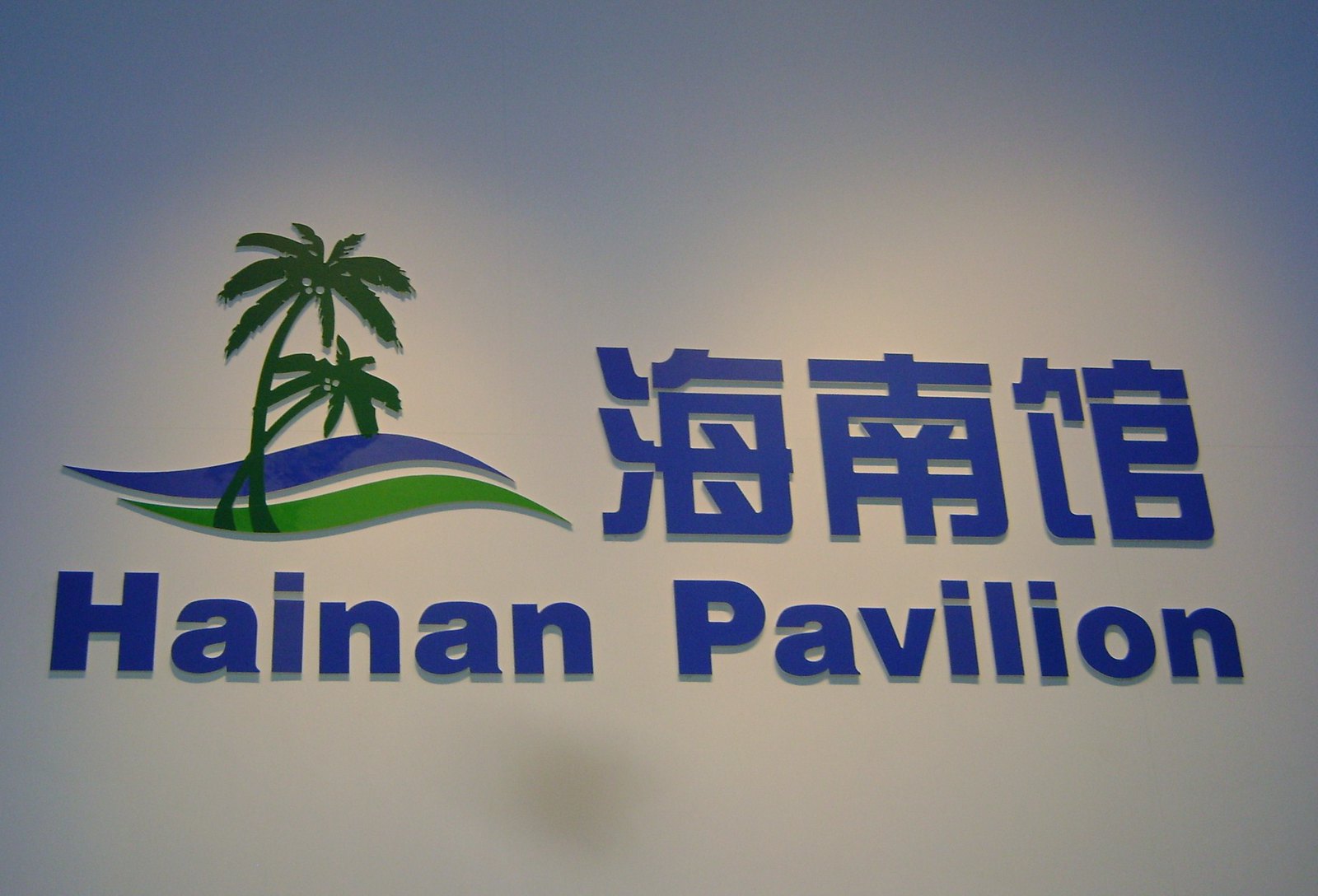This image showcases a prominent sign or logo attached to a white wall, possibly in a building or hotel. Dominating the left side of the sign are two green palm trees, one shorter and leaning into the other's shade. Beneath these palm trees are two wave-like lines, one blue and the other green, adding a touch of color and movement to the image. To the immediate right of the palm trees, three Chinese symbols are displayed in blue, contributing to the cultural theme. Below these symbols, the words "Hainan Pavilion" are elegantly written, also in blue. The sign sits against a background that fluctuates in color, blending shades of blue, light gray, and white, creating an interesting and dynamic backdrop for the logo. The design is large and centrally positioned within the photo, making it the focal point.